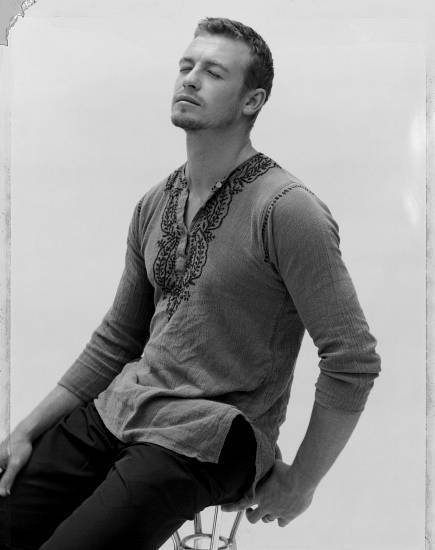This black and white studio portrait features a young Caucasian male, possibly in his early 30s, with short light brown hair. He is sitting on a bar stool with a base comprised of four metal rods, although the top of the stool is not visible. His eyes are closed, and his head is tilted back slightly, as if basking in sunlight. He wears a distinctive casual shirt with a v-neck, adorned with lace stitching along the collar and halfway down the chest. The sleeves of the shirt are rolled up to mid-arm. On his face, he sports a short goatee and a mustache akin to a Fu Manchu. He is dressed in what appear to be black jeans. The background is plain white, featuring some scratches or borders suggestive of a scan from a film negative or black and white slide, with additional highlights on the right side that could be due to a light leak or scanning error. The scene conveys a serene, introspective mood, enhanced by the monochromatic palette.